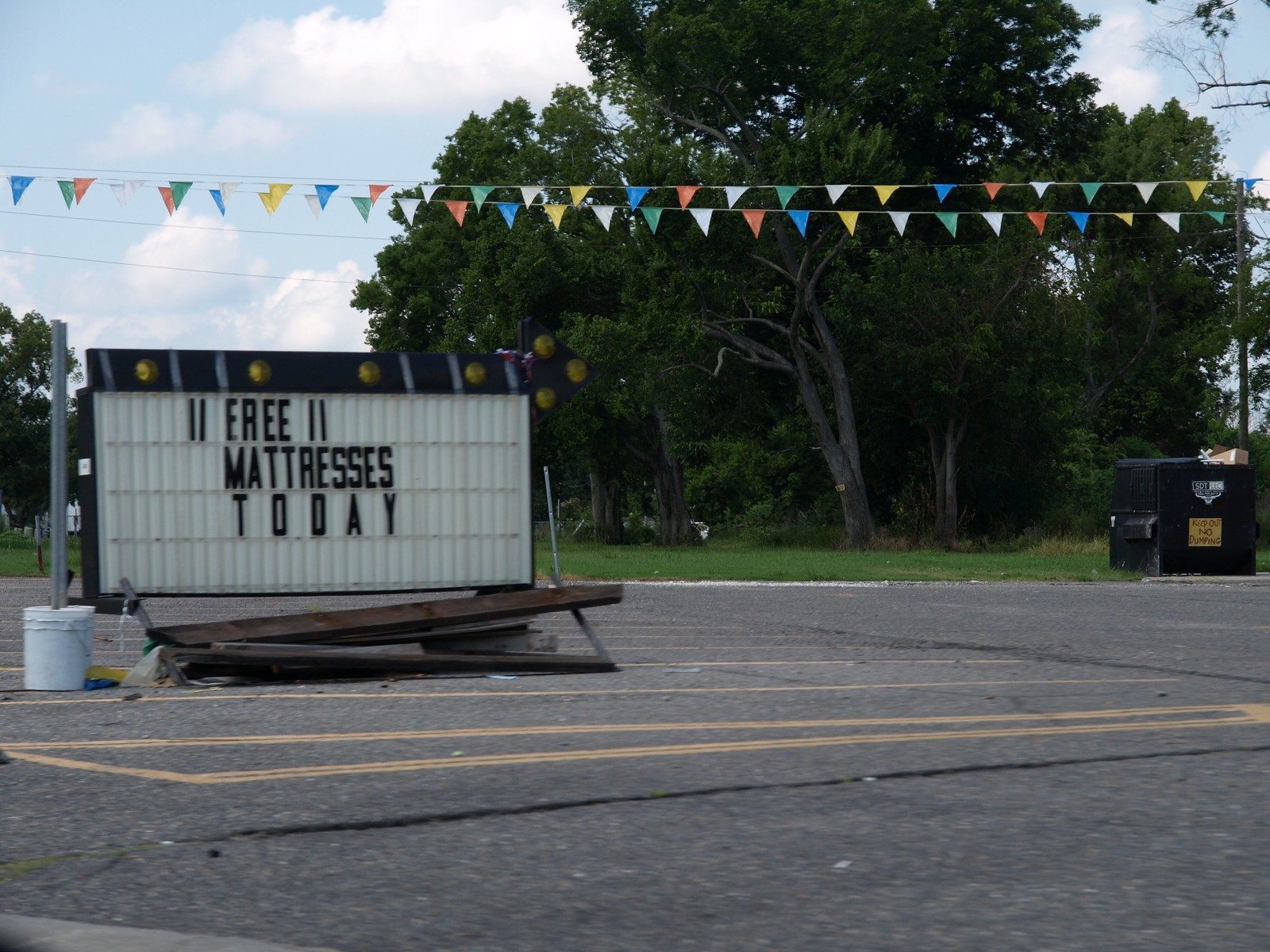The image depicts an empty asphalt parking lot on a daytime with partly cloudy skies. Prominent in the scene is a large promotional sign on the left side, featuring black letters spelling "Free Mattresses Today" on a white background. The sign is accompanied by scattered debris including some old wood and a white bucket. In the background, slightly towards the left, there's a sizeable green dumpster filled with trash, with large trees and grass beyond it. A power line pole stands behind a garbage can positioned at the bottom right of the image. Additionally, colorful triangular celebration flags hang from the posts across the parking lot, highlighting a possible sale or event. Yellow painted lines marking parking spaces can also be seen on the asphalt. The overall setting has an abandoned feel, with no cars present and an air of neglect.